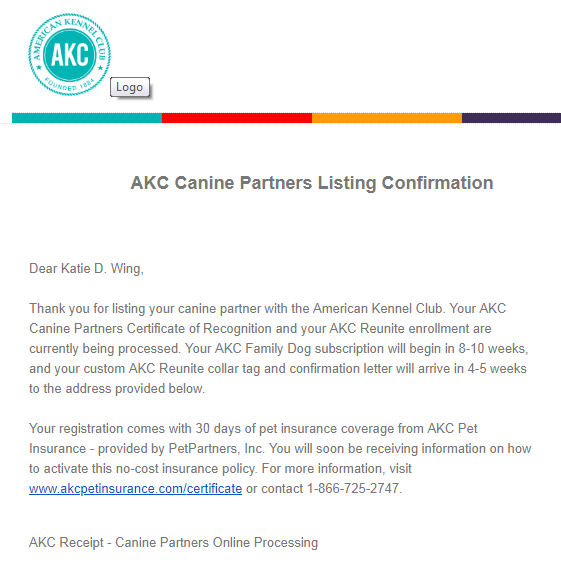The image showcases an official document addressed to Katie D. Wing from the American Kennel Club (AKC). The prominent AKC logo is displayed at the top, featuring a blue emblem with intricate detailing. Below the logo, a combination of red and yellow elements are visible, highlighting important information.

The document is a notification regarding the successful listing of Katie's K9 partner with the AKC. It acknowledges the ongoing processing of the IKC K9 Partner Certificate of Recognition and the re-enrollment procedures. The letter outlines that Katie will soon receive her IKC Family Doc subscription, which will commence in 10 weeks, and informs her about a renewed customer contact period of 4-5 weeks.

Additionally, the document details that Katie's address has been used to provide 30 days of free pet insurance coverage through IKC Pet Insurance, administered by Pet Partners Inc. Instructions for activating the insurance policy, including the website (www.ikcpetinsurance.com) and contact number (1-866-725-2747), are provided.

The entire document is set against a plain white background, emphasizing the text and logos for clarity.